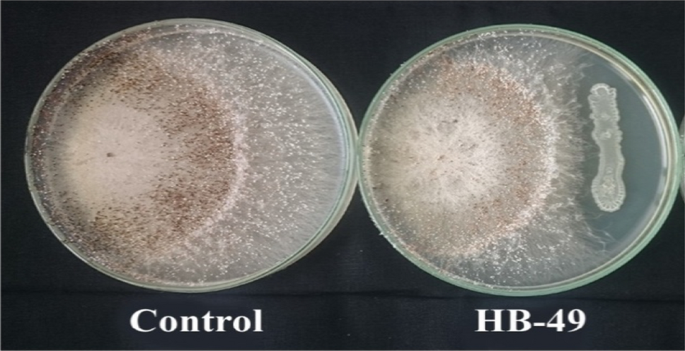The image displays two elliptical agar plates, each inset against a black background with white text labels beneath them. The plate on the left is labeled "CONTROL" and the one on the right is labeled "HB-49." Both captions are in uppercase letters.

The **control plate** on the left has a distinct radial structure toward its center. At its core, there's a small black dot surrounded by a light tan circle. This inner circle transitions into a darker brown outer ring, giving it a layered appearance. Encircling this brown ring, there's a thin white band along with numerous small white dots scattered towards the outermost area.

In contrast, the **HB-49 plate** on the right has a less defined center. The core is not as sharply marked as the control's, and its surrounding circle is whiter and appears rougher. The brown ring on this plate is lighter and less pronounced. Additionally, the plate contains fewer peripheral particles. Notably, on the far right side, there is a separate patch of whitish gel-like substance, with the small white dots kept at a distance from this area.

Overall, the image provides a clear visual comparison between the control and HB-49, highlighting differences in structure, pattern, and particle distribution. This scientific slide photo captures the detailed growth patterns of the organisms present on the agar plates.